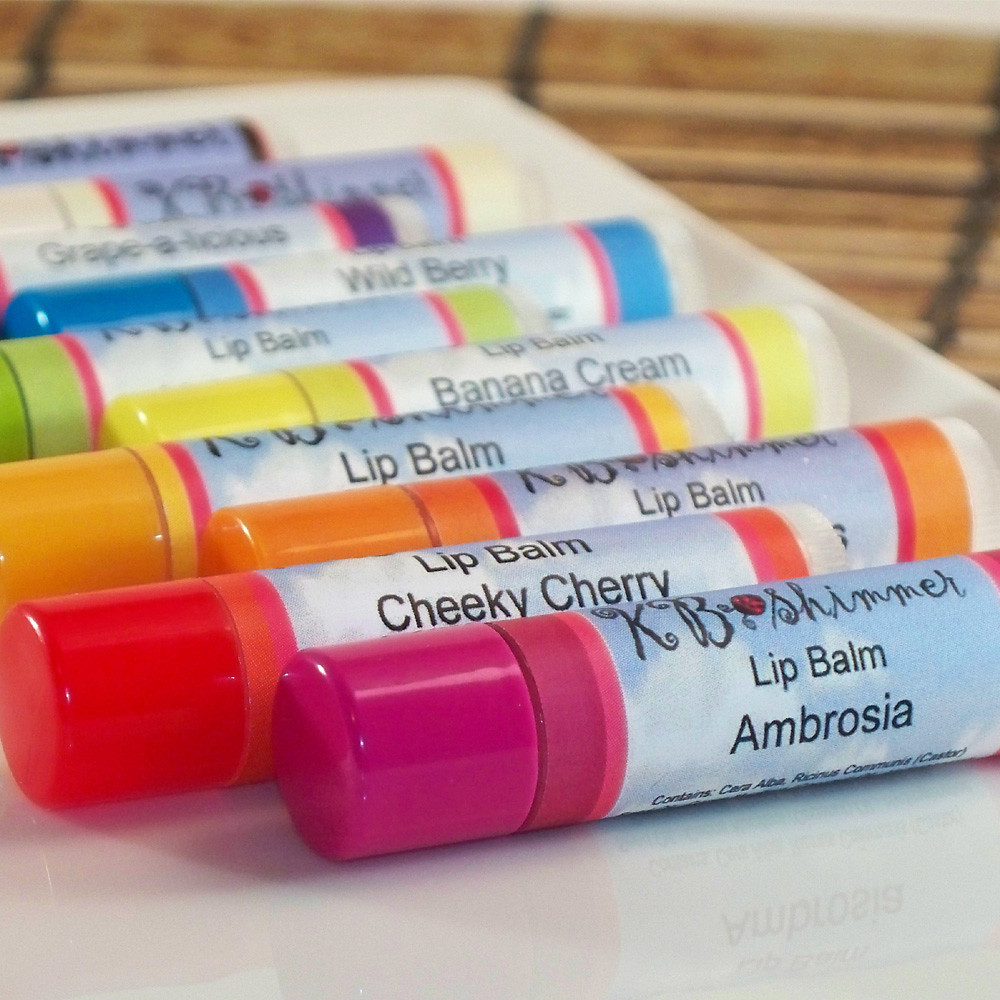In this detailed photograph, ten tubes of chapstick are meticulously arranged on a white surface, creating a colorful line that gradually blurs into the background. The chapsticks are distinguished by their vibrant caps, which come in a variety of shades including pink, red, orange, yellow, green, blue, and purple. Each tube is adorned with a clear label featuring a soothing blue sky and white clouds design. Prominently displayed in black text on each label is the brand name, KB Shimmer, along with the product description, "Lip Balm." Additionally, specific flavors are indicated, such as Ambrosia on the first tube, followed by Cheeky Cherry. Further back, we also see flavors like Banana Cream and Wild Berry. The background of the image reveals a blurred wooden texture, adding a subtle contrast to the colorful array of chapsticks in the foreground.